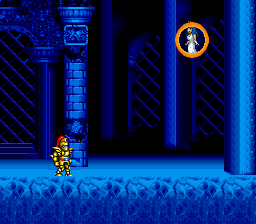In this striking video game scene, the environment features a dark bluish backdrop complemented by a stone-like textured floor. The ground is divided into two sections: the front part showcases a flat blue surface, while the area where the player character walks is positioned more to the left. The focal point of the image is a knight-like figure adorned in golden armor and equipped with a helmet. The character is depicted with long reddish hair flowing, gazing towards the right side of the screen. This knight is moving from the left side of the screen. Additionally, an orange-gold circle appears in the upper right corner, containing what seems to be a purse at its center, possibly indicating an in-game item or objective. The overall scene exudes a sense of adventure and fantasy, inviting the player into a meticulously crafted digital world.